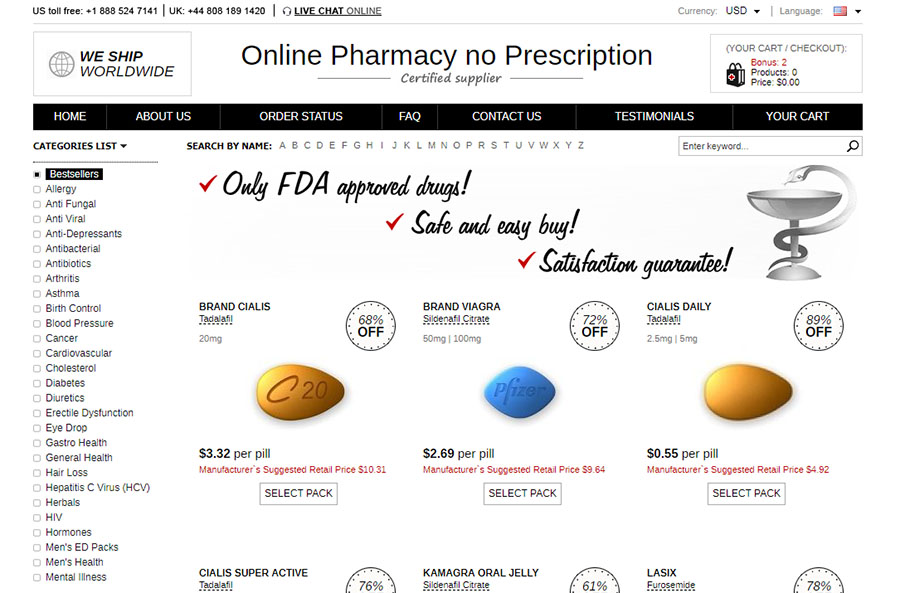This screenshot depicts an online pharmacy website. Dominating the top of the page in large font is the text "Online Pharmacy No Prescription." Centrally featured are images of three large pills: a yellow, egg-shaped pill marked with "C 20," a bright blue, diamond-shaped pill labeled "Pfizer," and another egg-shaped, gold-colored pill. In the upper right-hand corner, there is a shopping cart icon depicted as a bag within a rectangle, accompanied by text that reads "Your Cart, Checkout, Bonus Products, Price." A vertical menu runs down the left side of the page, while a horizontal menu spans the top. The pills are identified and priced as follows: Cialis at $3.32 per pill, Viagra at $2.69 per pill, and another variant of Cialis at $0.55 per pill.